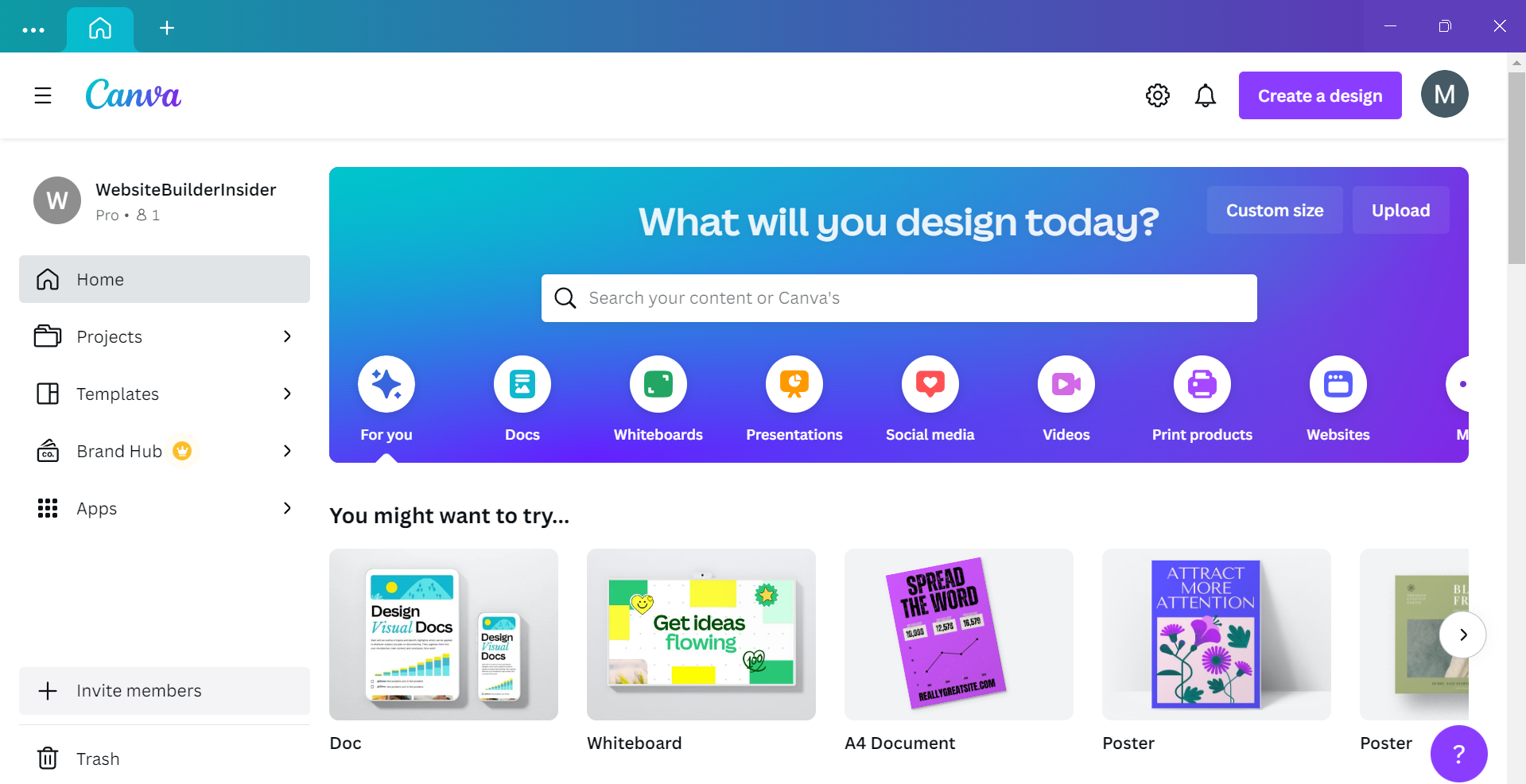This image depicts the Canva website interface. At the top, there is a vibrant navigation bar that transitions from turquoise on the left to purple on the right. On the far left of this bar are three ellipsis points, followed by a Home button with a Home icon, which is currently selected. Adjacent to the Home button is a white plus sign. 

To the far right of the navigation bar, there are three icons: a dash, what appears to be a coffee cup, and a white "X" in the top right corner. Beneath this navigation bar lies the Canva logo, also sporting the same turquoise-to-purple ombre effect. To the left of the logo, three dark gray horizontal bars signify the main menu.

On the right side of this secondary bar, icons for Settings, Notifications, and a purple "Create a Design" button are displayed. The user profile picture, depicted as a dark gray circle with an "M" in the center, is also located here.

The main content area of the website features the prompt, "What will you design today?" with options to search content or Canva templates. Various categories are listed below this text, including "For You," "Docs," "Whiteboards," "Presentations," "Social Media," "Videos," "Print Products," and "Websites." Suggestions like "Doc," "Whiteboard," "A4 Document," "Poster," and "Poster" are highlighted in white.

On the left side of the site, another menu is present, displaying the user's name as "Website Builder Insider," indicating they are a Pro user with one person on the plan. This vertical menu includes options for "Home," "Projects," "Templates," "Brand Hub," and "Apps."